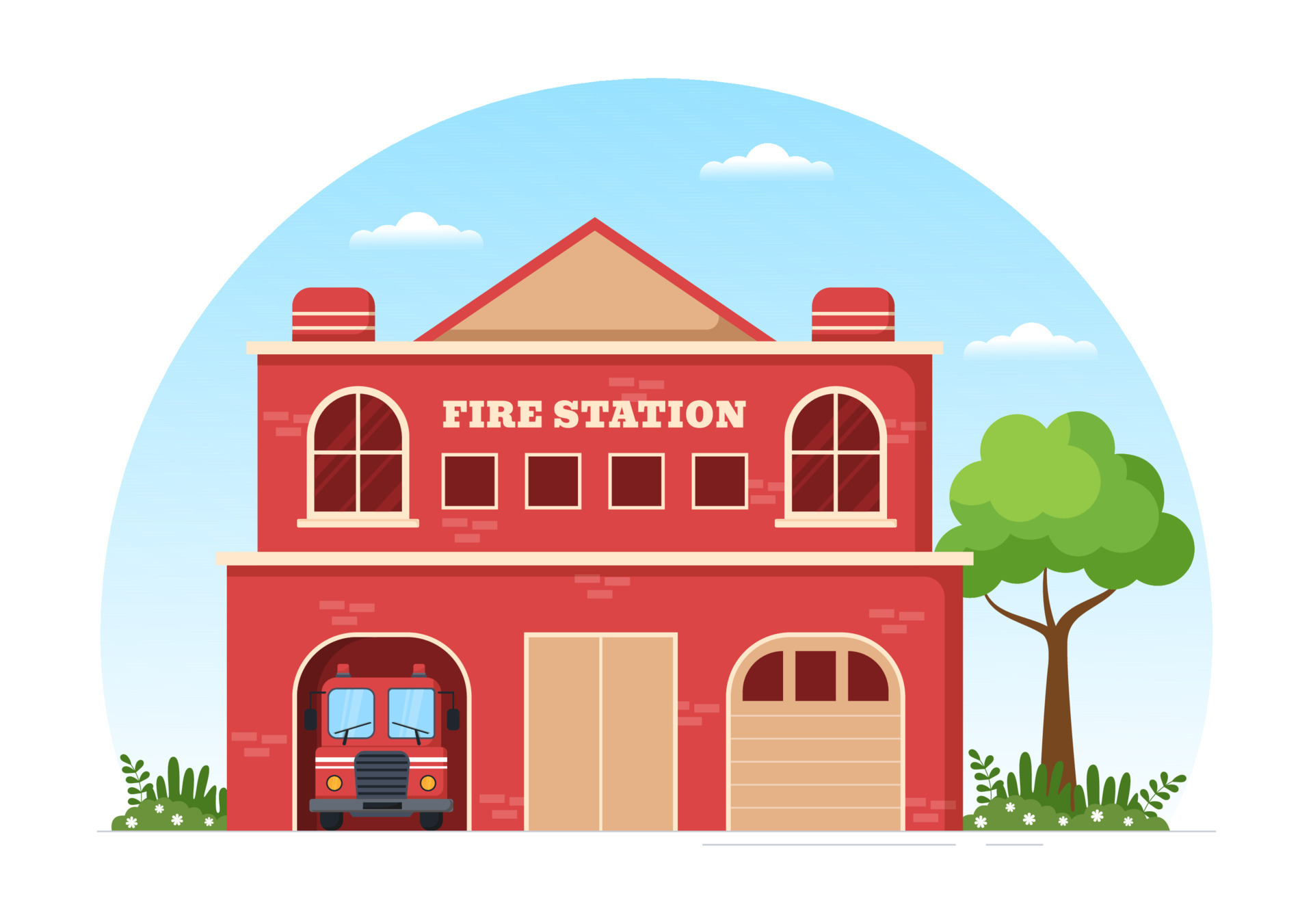This clipart image depicts a charming cartoon fire station set against a serene, bright blue sky with a few fluffy white clouds. The sky background forms a distinctive semi-circle or dome shape, framing the scene. The fire station, constructed of red brick, is the central focus and occupies most of the semi-circle border. It is a two-story building with a pointed roof and two chimneys, adding to its quaint appearance. The upper floor features prominent white lettering spelling out "Fire Station" and includes two sets of windows, each with four smaller panes between them.

On the ground floor, there are three main sections: on the left, an open garage door reveals the front of a red fire truck; in the middle, large light brown double doors; and on the right, a closed light brown garage door. Flanking the fire station are patches of green grass, with a vibrant cartoon tree on the right side, its height nearly matching that of the building. The entire composition exudes a playful yet detailed charm, capturing the essence of a sunny day at a friendly neighborhood fire station.